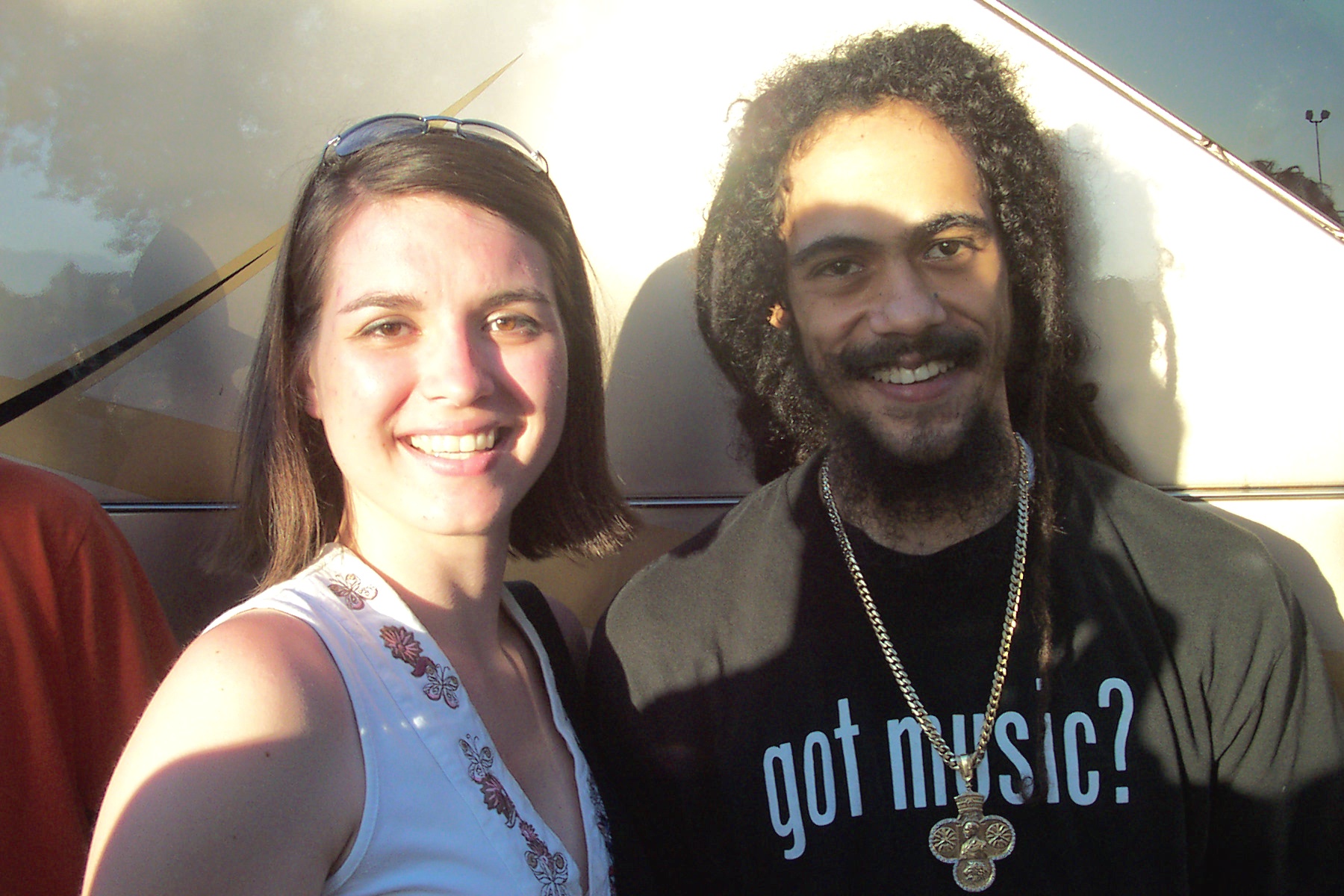In this outdoor photograph, a man and a woman stand closely together, posing for the camera. The background reveals elements of nature and a structure, featuring a portion of the sky, a tree, and a high light pole. You can see the edge of an A-frame building adorned with grey or tan, yellow, and black lines. 

The woman, positioned slightly to the left of the man but facing the camera, wears a white tank top with thick straps and a v-neckline decorated with embroidered red flowers and butterflies. She has short, dark hair and wears sunglasses perched on top of her head. Her expressive dark eyes gaze directly at the camera.

To her right stands the man, a black individual with curly hair that appears to be transitioning into dreadlocks, alongside a scraggly beard and a mustache. He sports a black long-sleeved shirt displaying the text "Got Music?" in white letters. Around his neck hangs a long gold chain with a medallion featuring intricate designs, including circular elements and potentially a depiction of a clover, a military figure, and a lion. 

Additionally, on the left edge of the photograph, only a partial view of another individual can be seen, identifiable by their orange shirt and partial shoulder and chest. The combined elements in the foreground and background create a scene of casual camaraderie in an outdoor setting.